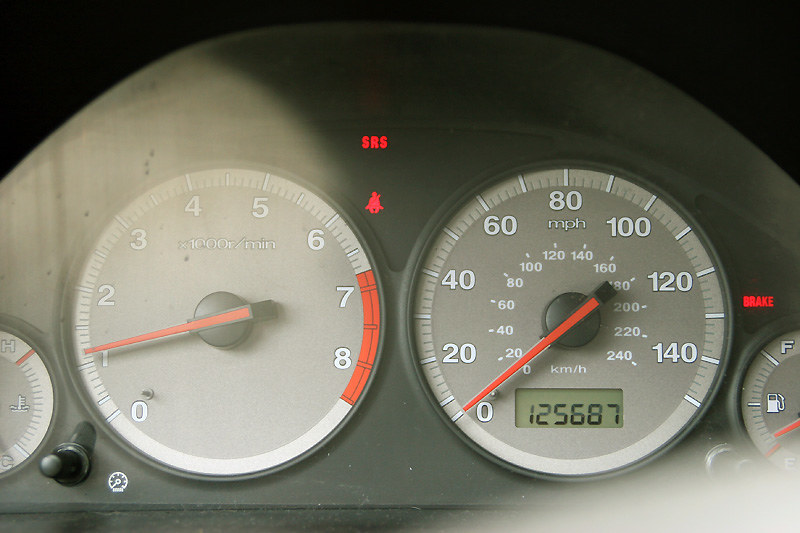In this landscape-oriented color photograph, the focus is on the dashboard of a vehicle, showcasing its detailed instrumentation. Dominating the image are two prominent, round gauges. Positioned on the right, the speedometer features a sleek gray face accentuated by crisp white numerals, ranging from 0 to 140. A vivid red arrow, anchored to a central dark disk, clearly indicates the current speed. Just above the lower edge of the speedometer, a small digital display reveals the vehicle's mileage, reading 125,687.

To the left of the speedometer resides another significant gauge, most likely a tachometer, which measures the engine's revolutions per minute (RPM). This gauge mirrors the design of the speedometer, with white numbers on a gray backdrop, stretching from 0 to 8. Notably, the segment between the numbers 7 and 8 is highlighted in bright red, indicating the engine's critical high RPM range. Both gauges share the characteristic red arrow mounted on a black disk at their center.

Centrally located between these two main dials, a small red warning light symbolizing the need for seatbelt usage subtly catches the eye, ensuring driver and passenger safety remains a visual priority. The interplay of colors and precise detailing of the dashboard's gauges provides a comprehensive and engaging depiction of this crucial vehicle interface.